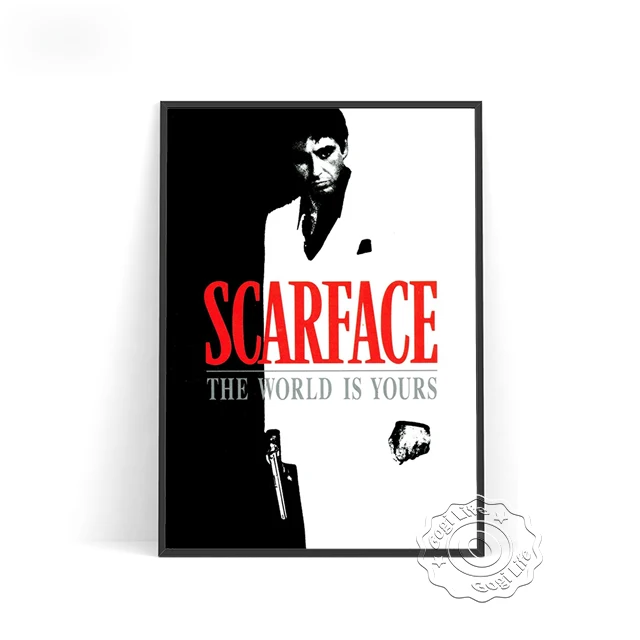The image is a striking black and white poster for the movie "Scarface" with bold red text at the top proclaiming the title "Scarface" and grey text below it stating "The world is yours." The image features Al Pacino as Tony Montana, positioned at the center and wearing a white suit jacket with a black shirt underneath, which matches the minimalistic, starkly divided black and white background. The left side of the poster is dominantly black, contrasting sharply with the almost entirely white right side, save for a handkerchief in the breast pocket. Tony Montana looks intensely serious with his dark hair framing his stern, angry expression. He holds a gun in his right hand, while a ring is visible on the finger of his left hand, which is clenched into a fist. In the bottom right corner, there's a watermark for "Gogi Life," stylized with an 'O' in the middle, resembling a flower pattern. This sophisticated poster oozes a minimalist and dramatic style, embodying the gritty essence of the film.